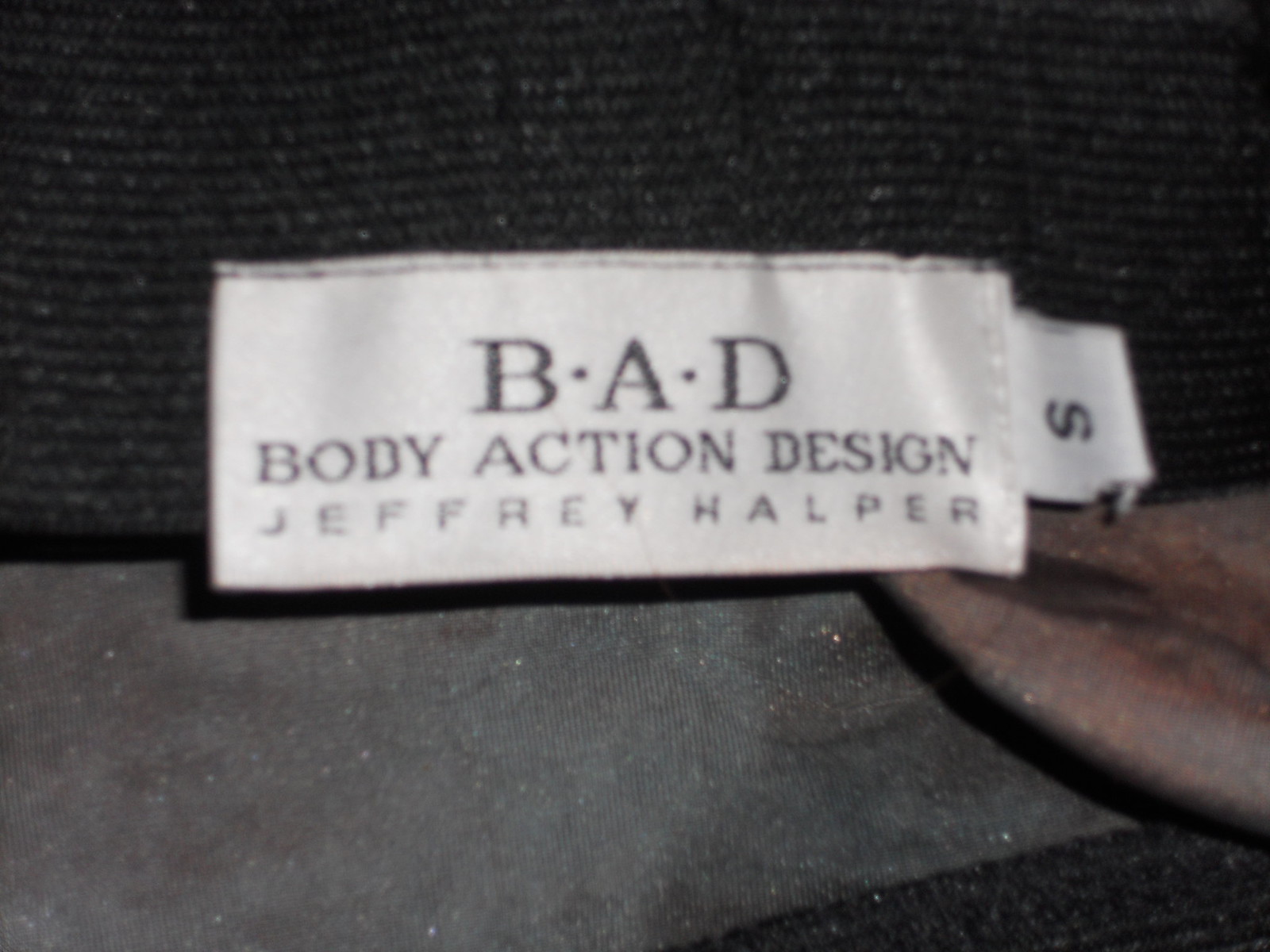The image features a close-up of a fabric with a label on the collar, which appears to be a thick, dark knit material transitioning to a lighter gray at the bottom. The top portion of the fabric is black with small white particles, while the bottom left section is a mix of gray and black. A brown object is situated on the bottom right.

Prominently displayed is a rectangular, white clothing label with black text. The label contains the following details:

- At the top, the label reads "BAD" where "BAD" stands for "Body Action Design."
- Below "BAD," the label states "Body Action Design Jeffrey Halper."
- To the right of this main label, there's a smaller, square tag, indicating the size "S" (small), with the "S" facing downward.

Although the item of clothing itself remains unclear, the detailed label strongly suggests it's a designer piece from Jeffrey Halper's Body Action Design line. The overall image is quite dark aside from the bright contrast of the white labels.